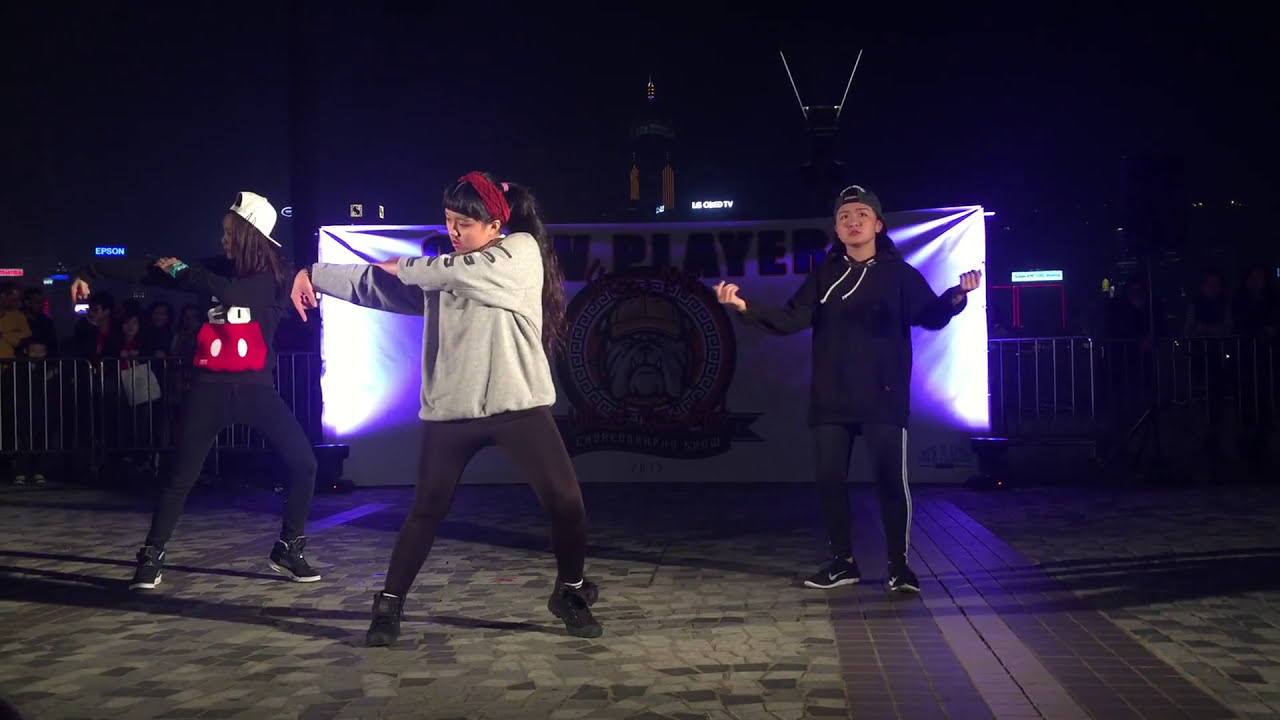In this nighttime outdoor scene, a color photograph in landscape orientation captures three adult women performing a hip-hop dance routine at the center of a public square or pavilion. The dancers are positioned on a gray cobblestone walkway, with two light panels on either side illuminating the area. The woman in the center, who appears to be the lead dancer, has long black hair, a red headband, a gray sweatshirt with writing on the sleeve, and black pants. Flanking her are two other dancers; the one on the right wears a dark sweatshirt with a hoodie, a backward black baseball cap, and black track pants with a white stripe. The dancer on the left wears a black sweatshirt, a white cap, and black tights. All three women have their arms outstretched in mid-move, adding dynamic energy to the scene.

Behind the dancers, a banner with an illustrated logo featuring a bulldog and the partially visible word "player" adds an element of intrigue, although the full text is unreadable. The background features a guardrail corralling a small crowd of onlookers, with a mix of neon signs and building lights punctuating the dark sky. The photograph, characterized by photographic representational realism, emphasizes the vibrant costumes of the dancers against the nighttime setting, with the majority of the image enveloped in shades of gray, black, and sporadic highlights of red, maroon, purple, yellow, and tan.